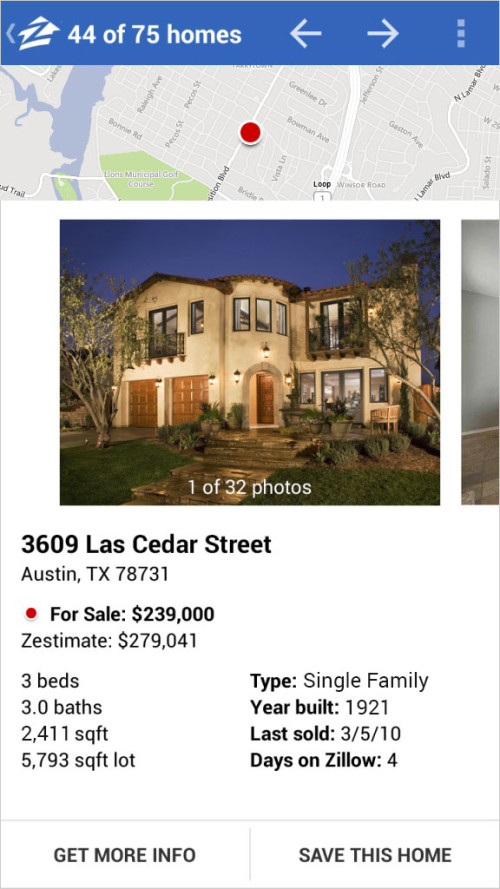Here is a cleaned-up and detailed caption for the described screenshot from the Zillow app:

---

The screenshot captures a page from the Zillow app. At the top, there is a dark blue navigation banner. On the left, a white arrow points left, next to the Zillow logo, which is a white house with a blue "Z" through the center. To the right, the banner displays "44 of 75 homes" in white text, flanked by larger arrows pointing left and right, indicating navigation controls.

Below the banner, the main section features a large rectangular map image with a red pin marking a specific location on a street. Underneath the map is a photo carousel box, starting with an exterior image of the house. The text "1 of 32 photos" in white appears at the bottom of the photo.

Beneath the photo box, the address of the house is displayed in black text. Following this, several details about the listing are provided: 
- "For Sale" status 
- The listing price 
- The Zestimate, or estimated value 
- House specifications, including three bedrooms, three bathrooms, total square footage, and lot size.

Additionally, on the right side, further information is presented: 
- The type of dwelling (single family) 
- The year the house was built 
- The last sale date 
- The number of days the property has been listed on Zillow.

At the very bottom of the page are two actionable buttons. The button on the left, "Get More Info," allows users to request additional details about the listing. The button on the right, "Save This Home," enables users to save the property to their favorites.

---